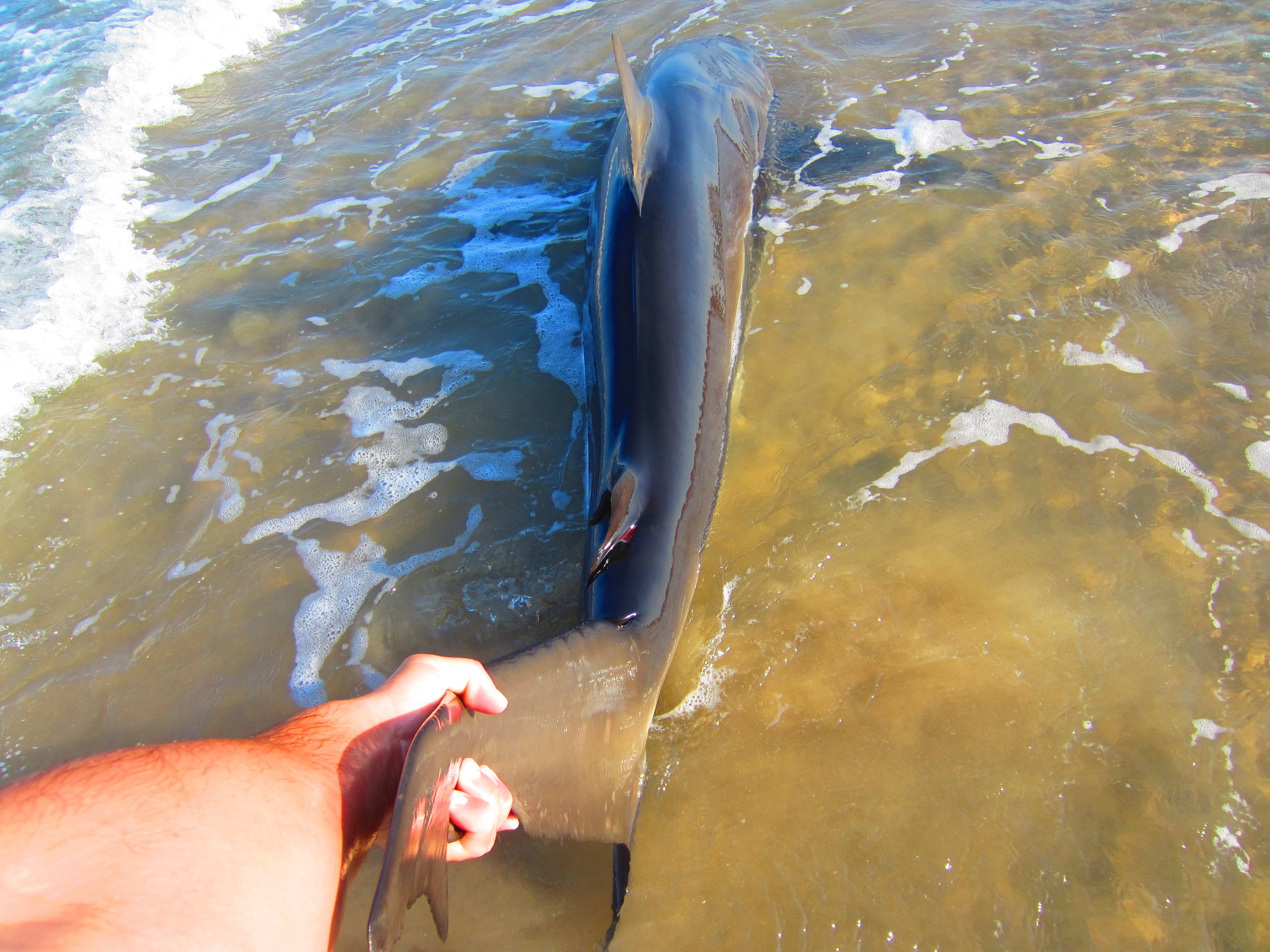In this image taken from a POV perspective, presumably with a GoPro, a man is standing at the edge of a beach, with his left arm clearly visible, extending to hold the tail fin of a large marine animal. The animal, which might be a dolphin, shark, or even a small whale, occupies almost the entire vertical span of the image and features distinctive gray skin with a prominent dorsal fin. The scene is set in very shallow water, which is quite murky and brownish near the shore but clearer farther out. The man’s forearm and some hair on his arm are visible, while waves from the left create splashes and foam in the water, suggesting movement and a dynamic environment. The shallow water allows the sandy bottom to be seen under the ripples, adding to the detailed beach setting.